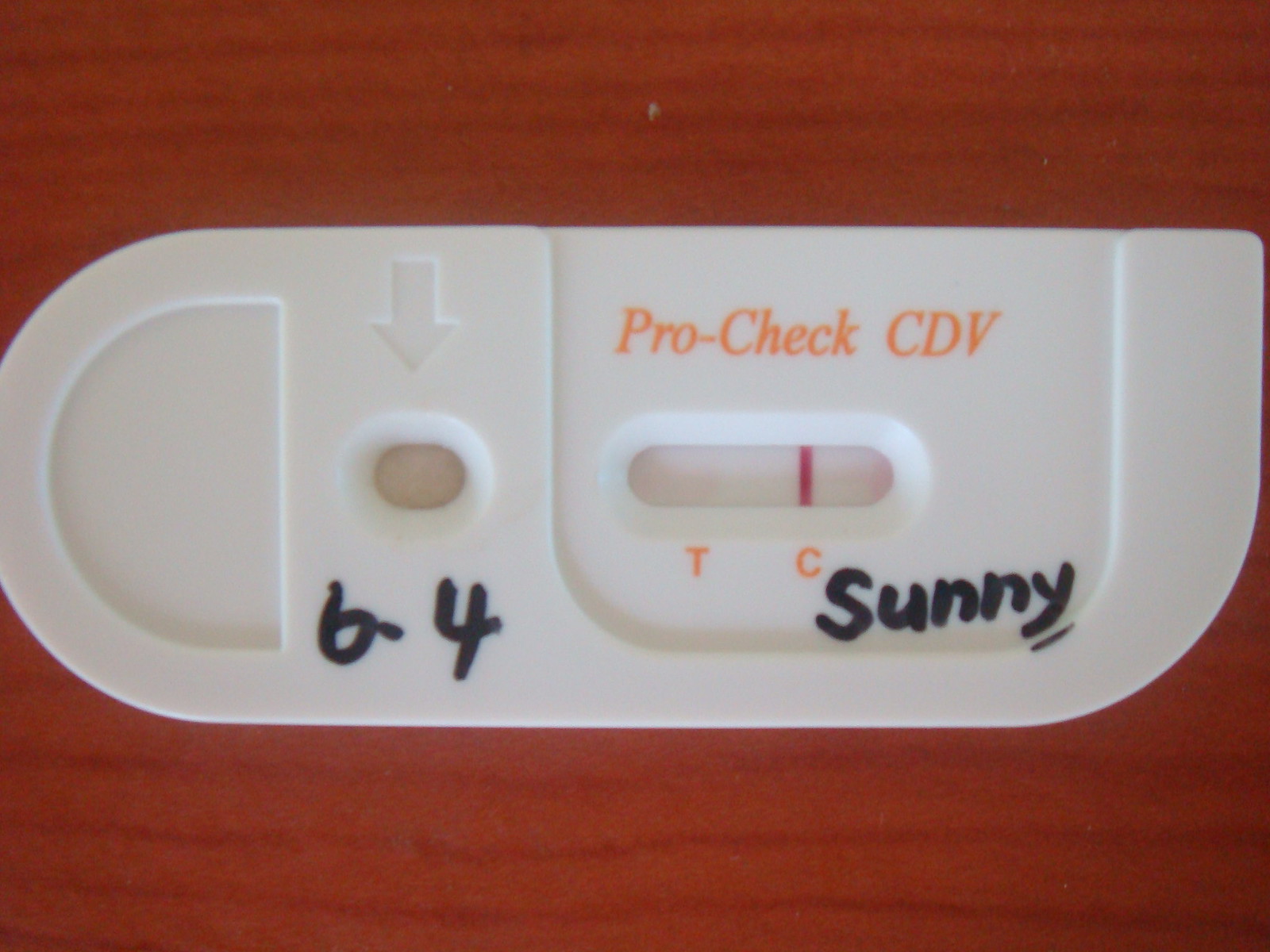The image showcases a close-up of a white testing strip, possibly for COVID-19, resting on a wooden table. The strip features a circular top and a flat bottom. Prominently labeled "PRO-CHECK® CDV," the strip has an arrow pointing to a small well, a divot situated in the lower section of the device. To the right of this well, there is another marking, with a 'T' on the right side and a 'C' on the left side. Above the 'C' well, a vertical red stripe is clearly visible. The strip is also marked in black ink with "B-4" and "SUNNY," with the 'Y' in "SUNNY" underlined. The wooden table beneath the strip has a small white dot, adding a minor detail to the setting.